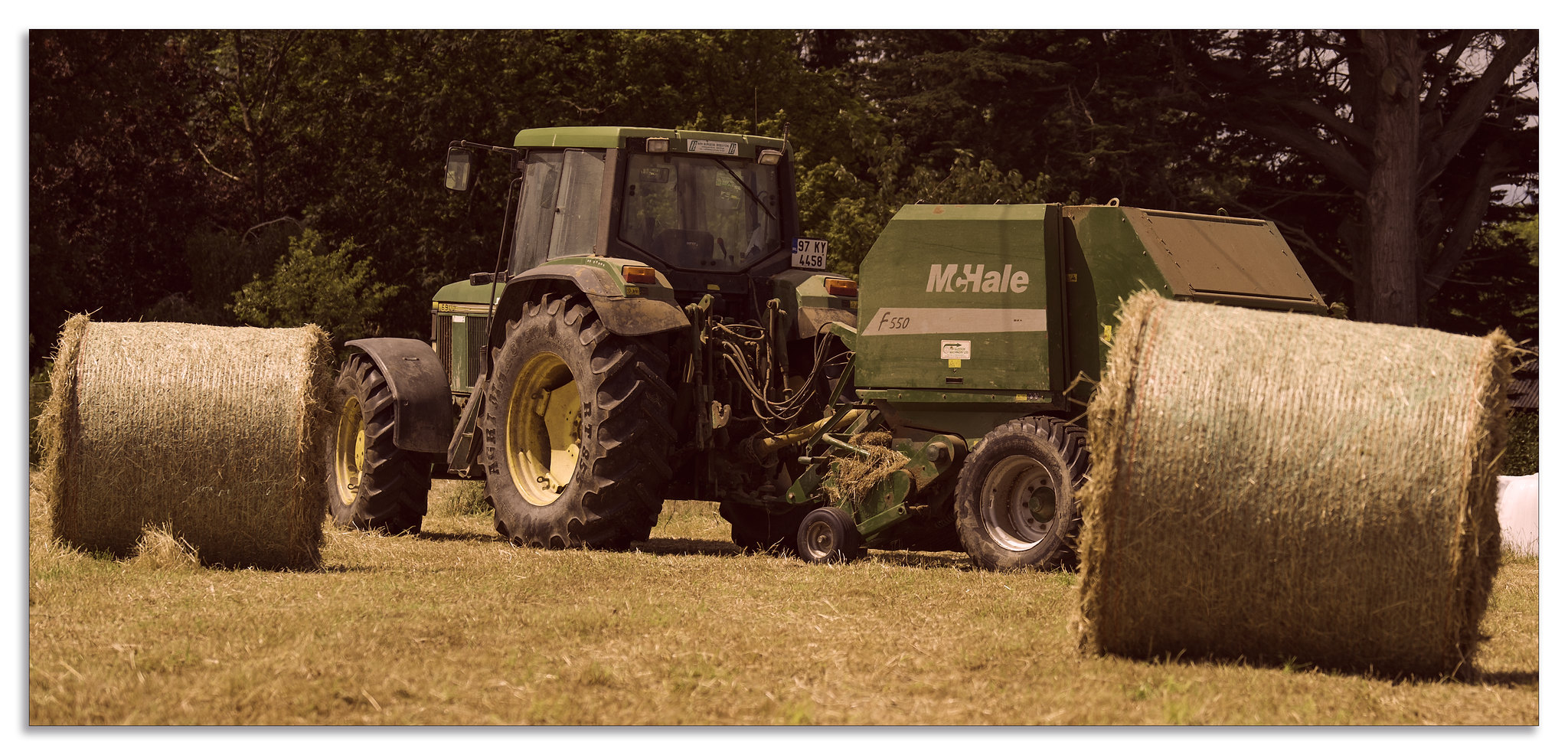This photograph, likely vintage due to a faded brown tint, captures a green McHale tractor stationed on a brownish grassy field, typical of a well-maintained farm area. The large tractor, viewed primarily from a rear-side angle, features towering black wheels, larger at the back than the front. Attached to the rear is a green box-like component bearing the white McHale logo, distinguished by a matching green "C." In front of the tractor lie freshly harvested hay bales, rolled into neat cylinder shapes, indicating that the tractor has recently been at work, possibly as a hay baler. Surrounding the scene are trees and foliage, adding to the rural atmosphere, with a glimpse of sky visible in the upper right corner. The image's overall vintage quality enhances the pastoral and historical feel of the setting.